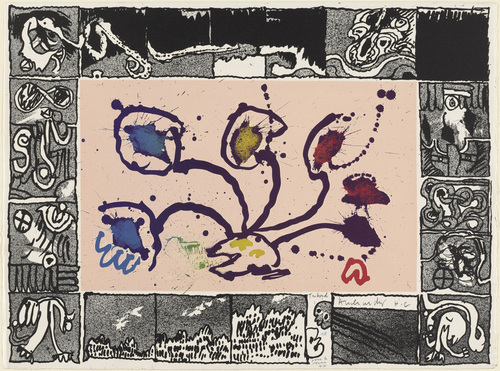The image is a wide rectangular artwork that resembles a painting. It features a beige-colored central section with a stylistic impressionist design of a plant. The plant has seven flower-like elements with deep purple semicircular stems that fan outwards. The flowers are distinctly painted with two on the left in blue, one in the middle in yellow, and four on the right in red. Surrounding this central motif is a border of black tiles, which is itself encased by a larger border of grayish beige. The outermost border is composed of 20 small squares that resemble cartoon drawings or scenes. These squares are black-and-white and vary in their illustrations, with some depicting abstract squiggly lines, faces, trees, and sky elements. The arrangement of the border is reminiscent of a Monopoly board, providing a frame of interconnected scenes that add a distinct and intricate context to the central plant design.